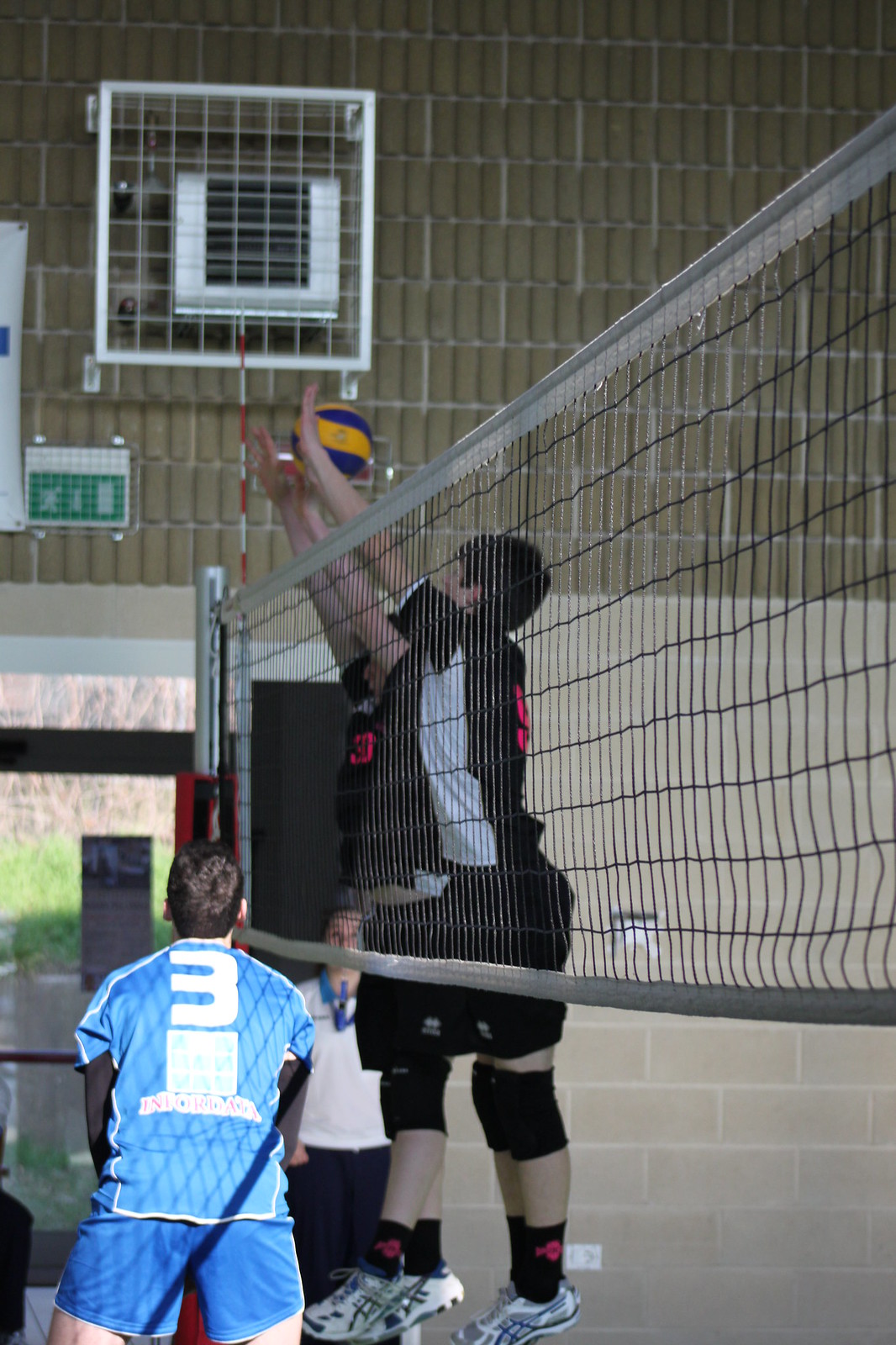This photograph captures an intense moment in a gymnasium volleyball match. At the center of the image stands the gray and black volleyball net, dividing the scene. On the left side of the net is a player wearing a blue jersey and shorts, with the number 3 and an indistinguishable logo in white text on the back. This player, who has fair skin and short dark brown hair, stands with arms extended in front of him and looks away from the camera, seemingly having just set up the ball.

On the right side of the net, two players in matching black, red, and white uniforms are captured mid-jump, with both feet off the ground and hands reaching over the net towards a yellow and blue volleyball. These players also have fair skin; the closer player has dark hair while the other's hair isn't visible. They sport coordinated black and white sneakers. The action unfolds in front of a gymnasium wall, whose lower part is white stone, contrasting with the yellow and white lines at the top. A black and silver air conditioning unit is mounted near the upper portion of the wall, adding to the detail of the indoor setting.